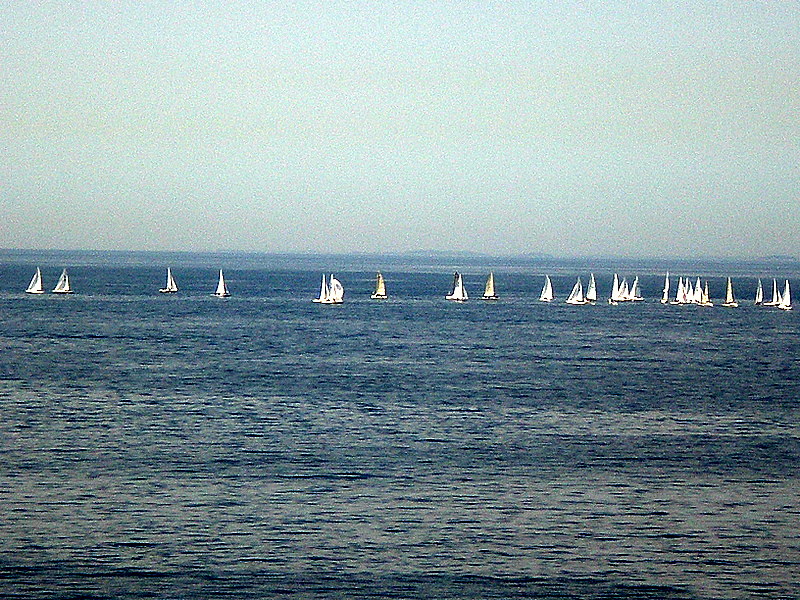The image captures a clear daytime scene of a large body of water, most likely the ocean, stretching out to the horizon where it meets a light blue sky. The water is bright blue near the horizon and transitions to a lighter, almost white hue near the bottom of the image. Central to the photograph, extending from left to right, is a distinct, uninterrupted row of approximately 15 small, white sailboats. Each boat's triangular sails are fully hoisted, suggesting they might be preparing for a race or are part of a coordinated search effort. The sailboats are lined up so precisely that they form what appears almost like a wall on the water, and they seem to be quite far from the observer, giving an expansive view of the scene. The photo, while clear in detail, also hints at a slightly misty or foggy atmosphere, with subtle indications of potential storm clouds in the distance, adding a touch of impending weather drama to the tranquil seascape.